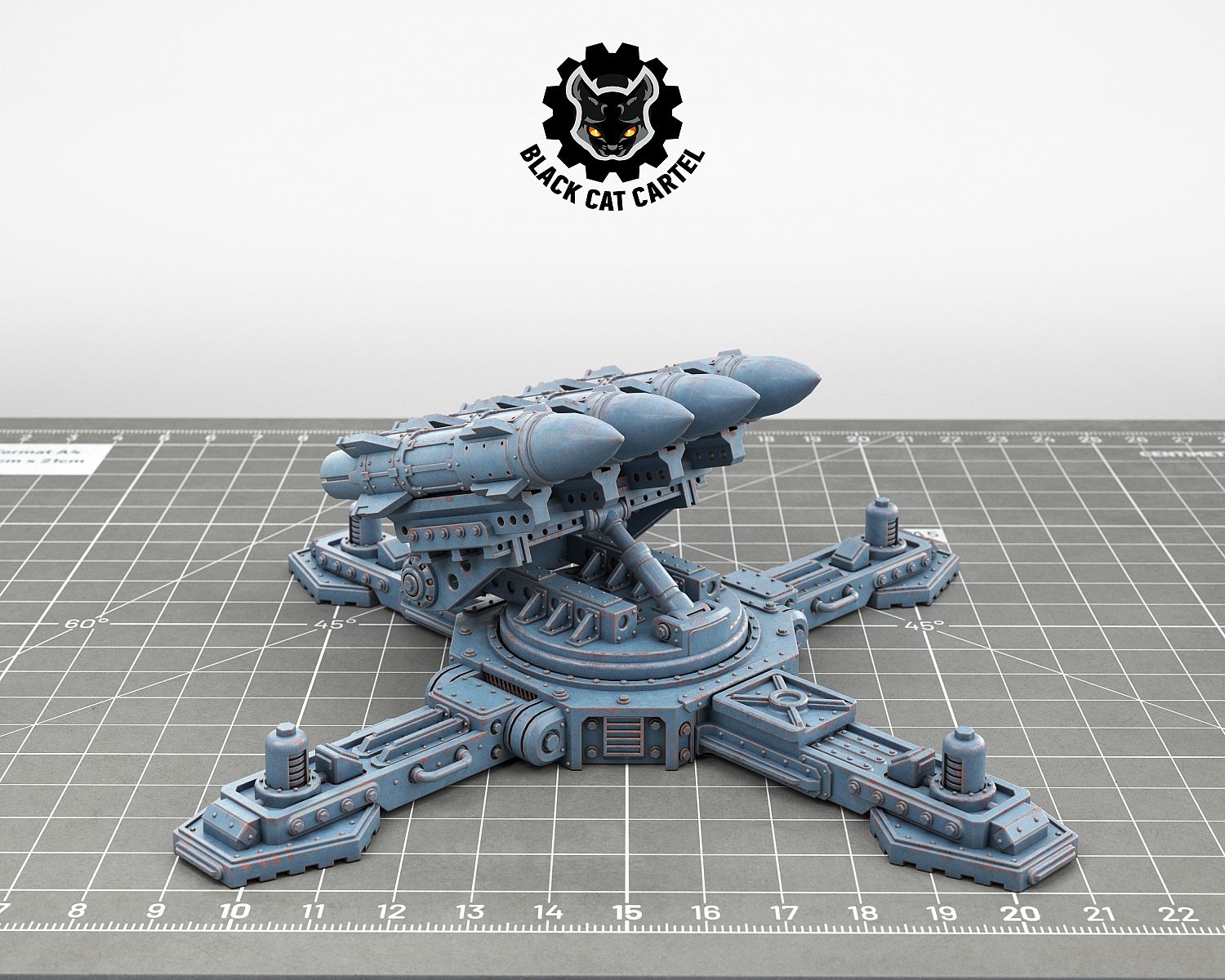This detailed photograph features a scaled-down model of a missile launcher positioned on a gray architectural cutting mat, marked with white measurement lines and numbers ranging from 7 to 22 centimeters. The launcher itself is a light bluish-gray color and consists of a crisscross type structure with four missile-like objects ready to launch, aimed upwards to the right. At the top of the image, there is a white background displaying an artistic, almost cartoony black cat's face encased in a black gear. The cat's face has glowing orange and yellow eyes and underneath this logo, it reads "Black Cat Cartel" in black letters. The grid lines on the mat and the detailed measurements, showing the launcher spanning from 9 to 21 centimeters and taking up about 12 centimeters horizontally, emphasize the precision and scale of the model.